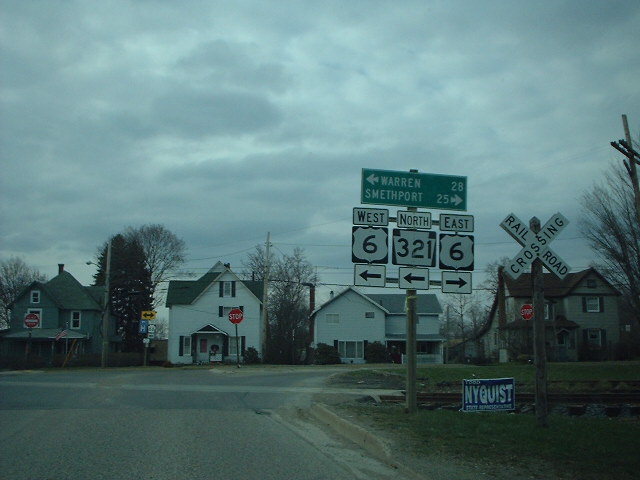This photograph captures a dreary, overcast day at a bustling intersection adorned with an array of road signs. The sky is dominated by thick, fluffy gray clouds, setting a somber mood over the scene. The intersection features a stop sign at the forefront, while a nearby railroad crossing sign marks the location of the train tracks just before the junction. Prominently displayed is a large green directional sign indicating distances and directions: 28 miles to Warren to the left, and 25 miles to Smethport to the right. It also details that West Highway 6 and North Highway 321 are to the left, while East Highway 6 is to the right. Below this, a blue and white Nyquist campaign sign is visible. The road, paved with macadam, stretches straight ahead and then curves to the right, flanked by various houses. On the left, a white two-story house and a gray-brown two-story house both have stop signs in front, while a smaller white house with a picket fence stands alone without any signs. Trees and bushes dot the landscape between these buildings, adding a touch of greenery to the scene.